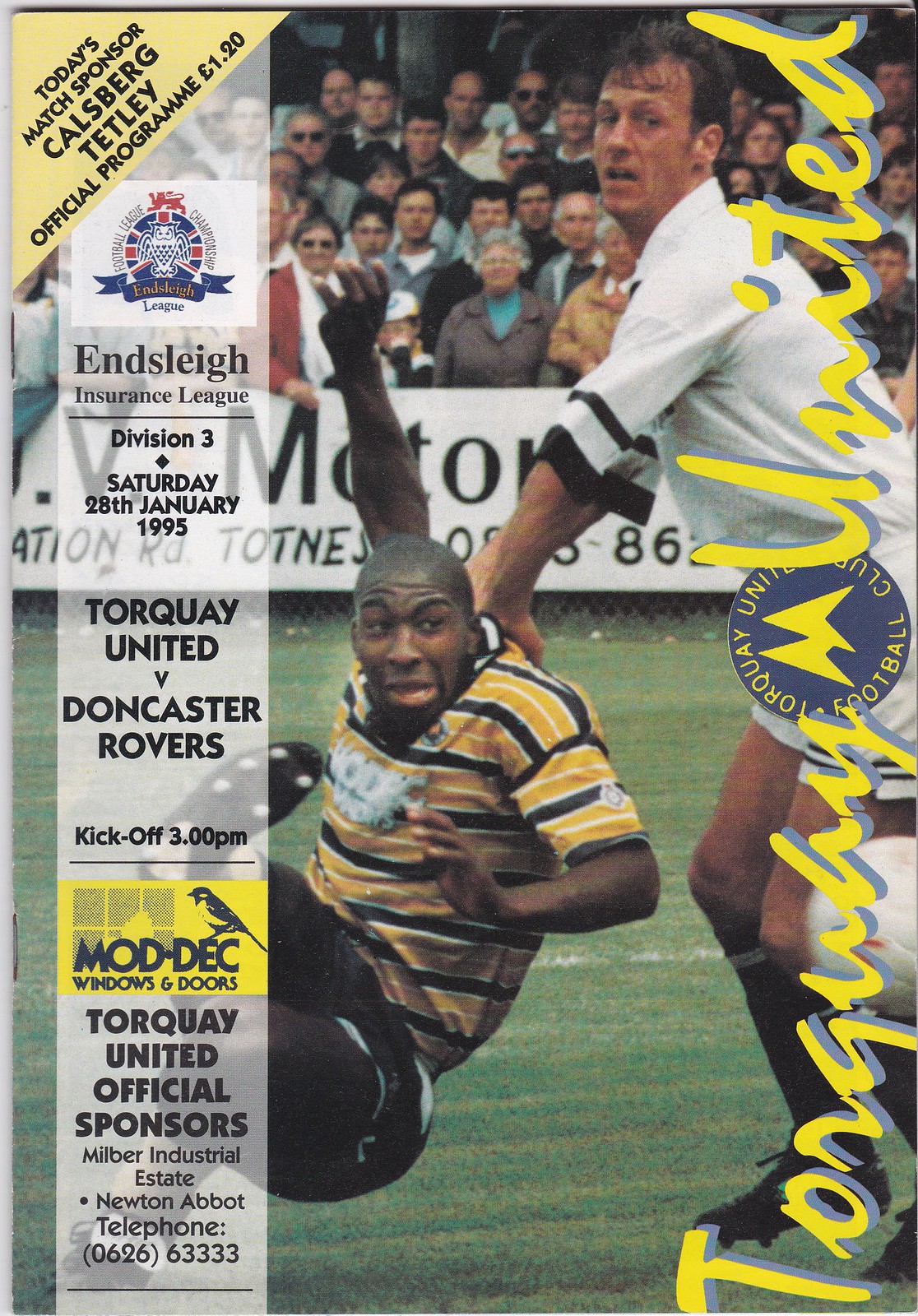This grainy photo from an official soccer program cover, dated January 28, 1995, for the Ensley Insurance League, Division 3 match between Torquay United and Doncaster Rovers, features a dramatic moment between two players. The player on the left, a black man in a yellow, black, and white striped shirt, appears to be mid-fall with his arms raised and white cleats visible. His expression is one of frustration. The player on the right, a white man dressed in a white uniform, has his hands on the back of the falling man's shirt, possibly contributing to his fall. Surrounding the image, there is text detailing today's match sponsor, Kalberg Tetley, the program cost of 1.20 euros, and additional sponsor information, including "Millburn Industrial Estate, Newton Abbott" and a contact number. The right side features a yellow cursive overlay reading "Torquay United," with a blue circle in the middle labeled "Torquay United Club Football." An advertisement for Modic Windows and Doors, characterized by a yellow background and a bird perched on the 'E' in Modic, is also present.